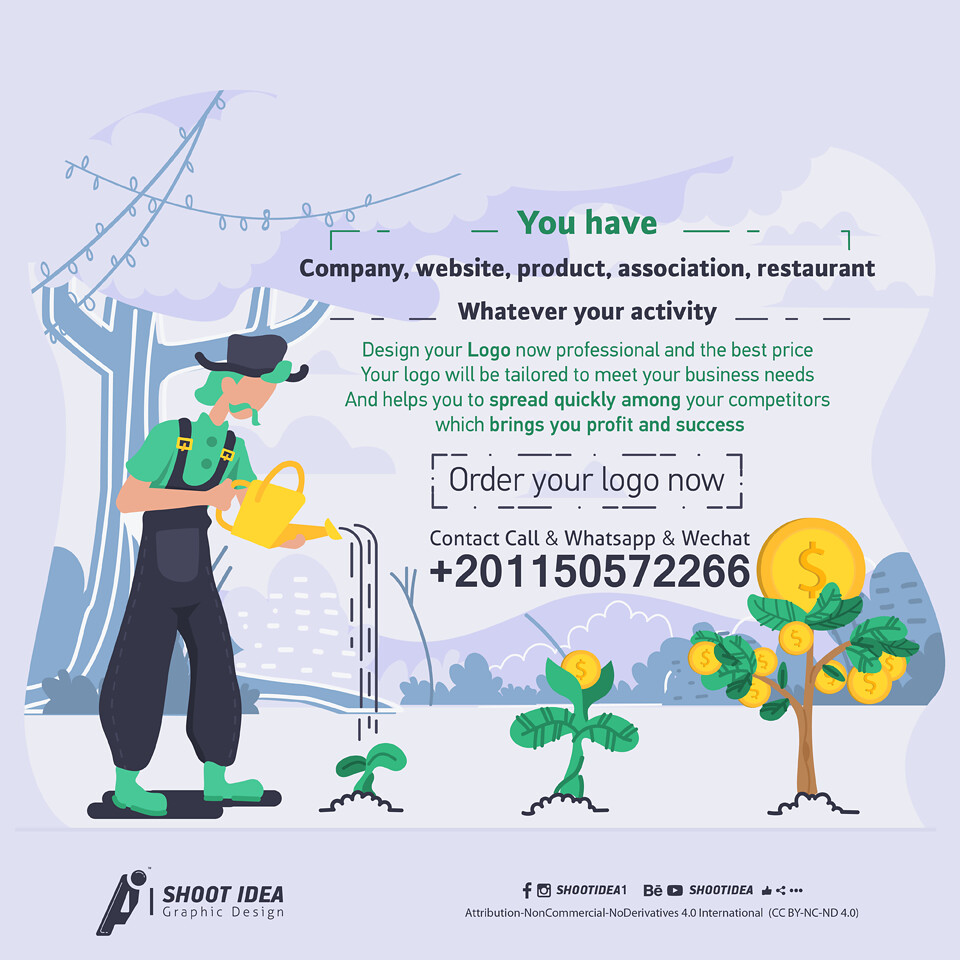The advertisement features a vibrant, cartoon-style design with a light purple background and a bold title that reads, "You have company, website, product, association, restaurant, whatever your activity." At the center-left of the image, a whimsical figure dressed in a green polo shirt, coveralls, green boots, and a black tall hat with green hair and a green mustache is watering three plants; the plants are arranged from shortest on the left to tallest on the right. Notably, the shortest plant being watered by the man is sprouting yellow coins with dollar signs symbolizing financial growth. Behind the man is a striking blue tree, adding a unique pop of color. Below the main illustration, details of the company "Shoot Idea Graphic Design" are provided, including a prompt to "Order your logo now" with contact information, phone number (201-1505-72266), and social media handles. The ad emphasizes creating a tailored logo that meets business needs, ensuring it spreads quickly among competitors, promising profit and success.